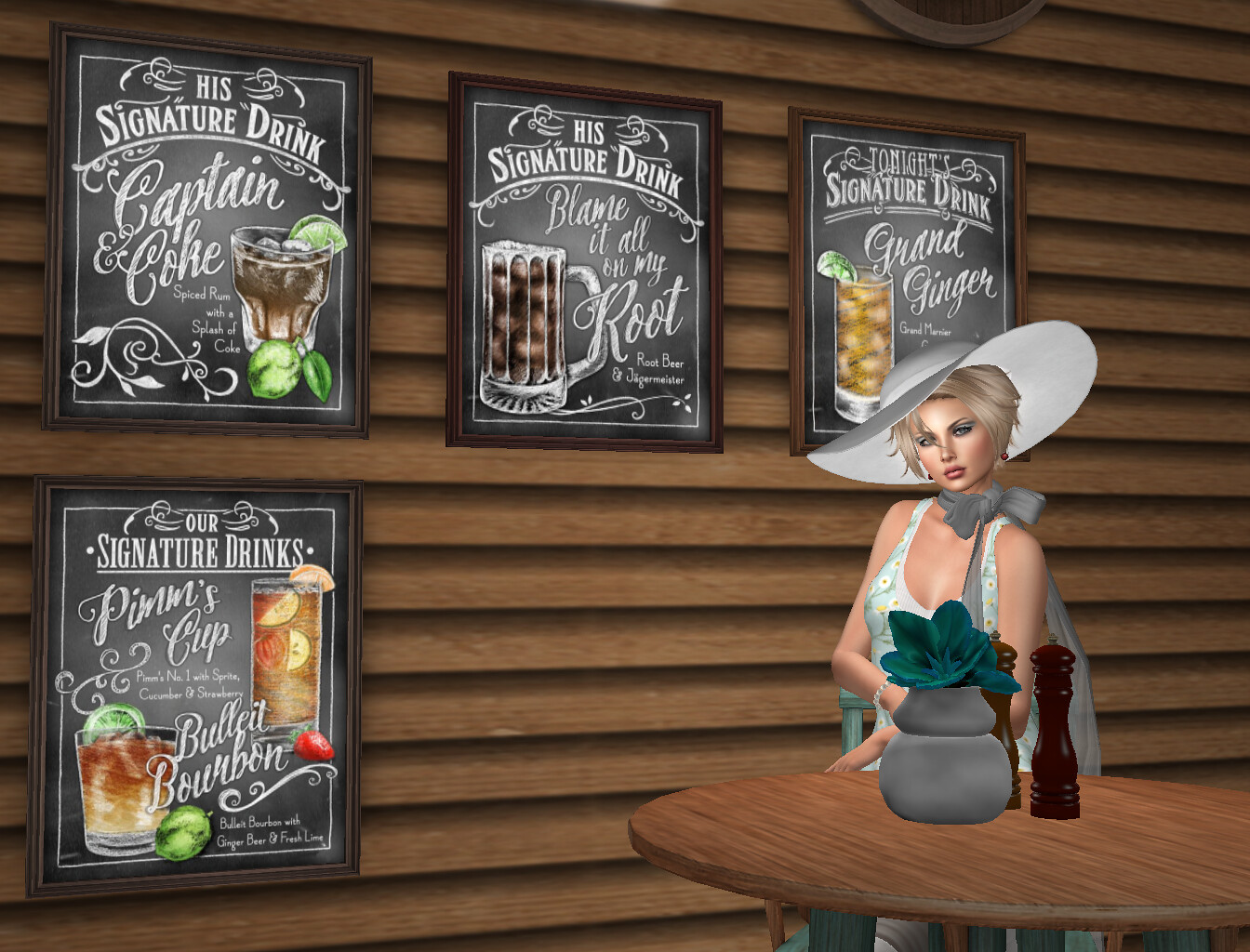The image is a computer-generated cartoon depiction set inside a restaurant or bar with a log cabin ambiance, characterized by a wooden clapboard and a slatted brown wall adorned with signs listing signature drinks: Captain Coke, Blame It All On My Root, Grand Ginger, Pins Cup, and Bullet Bourbon. In the bottom right corner, there's a wooden table featuring tall, wooden, twist-operated salt and pepper shakers and a ceramic vase with a green plant. A woman, leaning on this table, is prominently featured. She’s wearing an elegant wide-brimmed white hat and a sleeveless light blue tank top adorned with white daisies. She accessorizes with a gray bow tied around her neck and a diamond-like bracelet on her wrist. Her white-blonde hair complements her heavy makeup, which includes blue eyeshadow and small but thick lips, though she is not smiling.